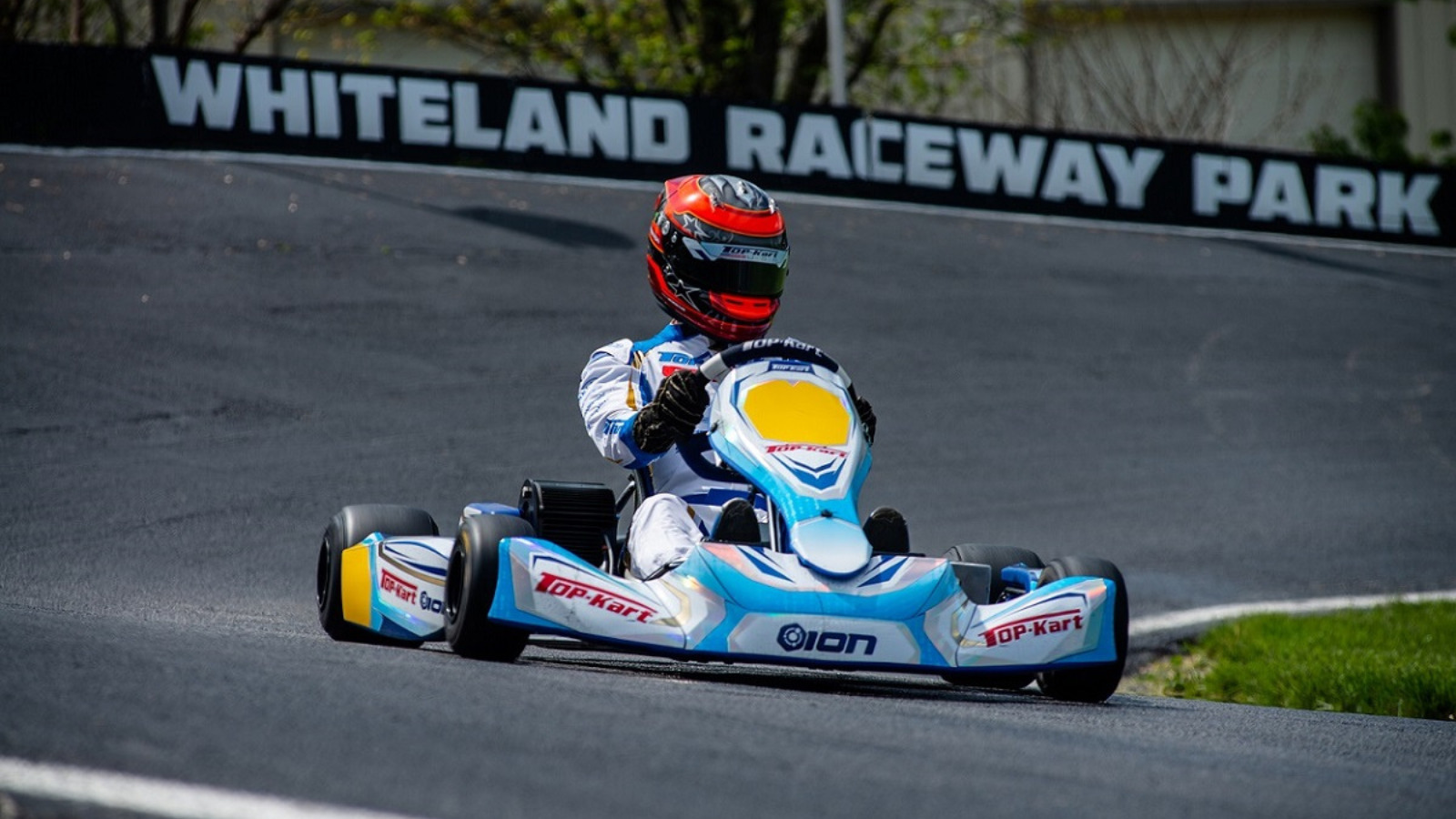In the image, a man is captured mid-turn racing a go-kart on the black asphalt track at "Whiteland Raceway Park," indicated by the large white letters on the black border surrounding the racetrack. The racetrack features white lines, and there is a spot of grass visible at the center of the turn. 

The go-kart driver is centrally positioned and wears a striking ensemble: a blue and white race suit, black gloves, and a red and black full-face helmet with a dark-tinted visor, obscuring his face. The go-kart itself is predominantly blue and white, featuring the words "Top Cart" on both the left and right near the wheels, with "Ion" written in the center. Additional details include yellow markings on the back fenders and on the steering column. The black tires of the go-kart appear smooth, and you can catch a glimpse of the driver's feet on the pedals as he navigates the turn.